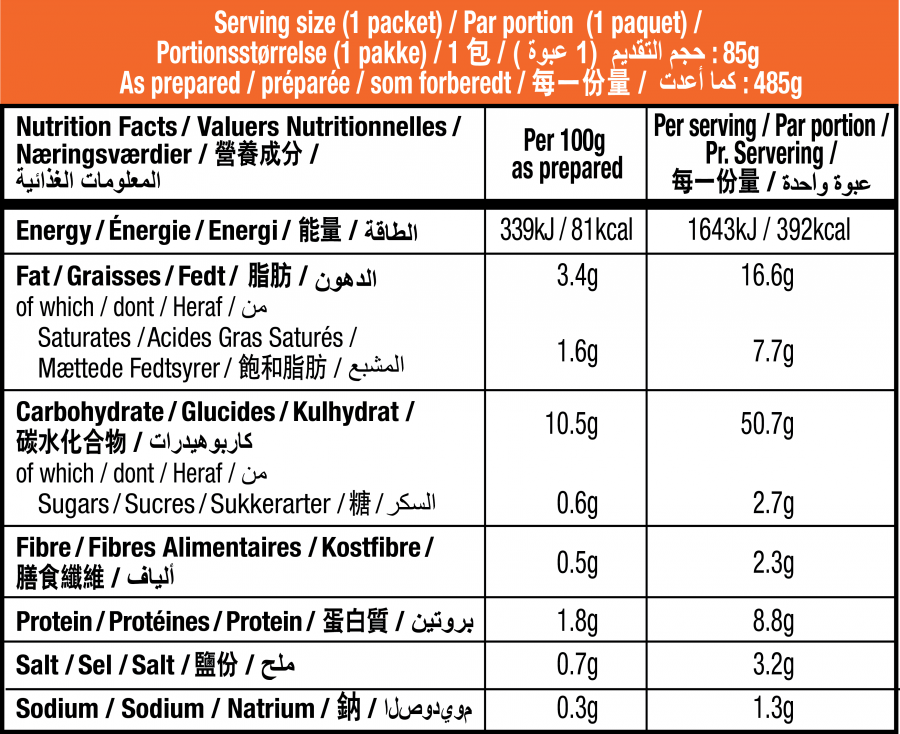The image depicts a detailed food package nutrition label with the top portion colored in orange and the majority of it in white with black borders. The label presents information in multiple languages, including English, French, German, Japanese, Arabic, and possibly Spanish. It prominently features standard nutritional details such as "Serving Size: One Packet," "Nutrition Facts," "Energy," "Fat," "Carbohydrates," "Fiber," "Protein," "Salt," and "Sodium." For example, the energy value is listed as 339 kilojoules / 81 kilocalories per 100 grams as prepared. The label comprehensively details nutritional values per 100 grams and per serving.